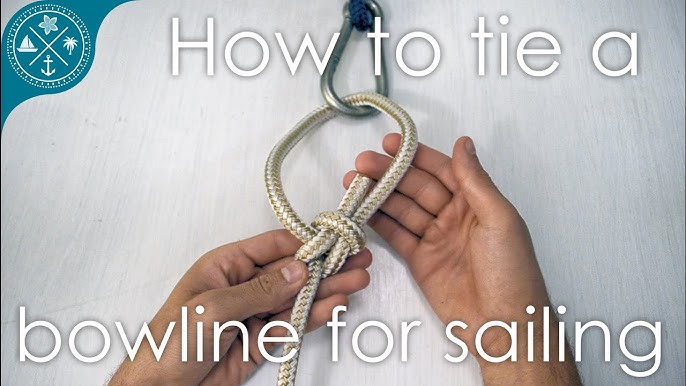The image depicts a detailed scene of a person tying a bowline knot on a whitish-goldish rope attached to a silver metal hook or buckle. Central to the image are the individual's hands in the process of knotting, with the bowline knot clearly showcased. Prominent white text spans the top and bottom of the image, boldly stating, "How to Tie a Bowline for Sailing." In the upper left-hand corner, a circular logo featuring a sailboat, an anchor, a palm tree, a star, and a flower is visible, suggesting a company or sponsor connected to the content. The background, with shades of grey, might be a wooden surface or fabric. The image is rectangular, and the meticulous knotting process stands out as the primary focus.